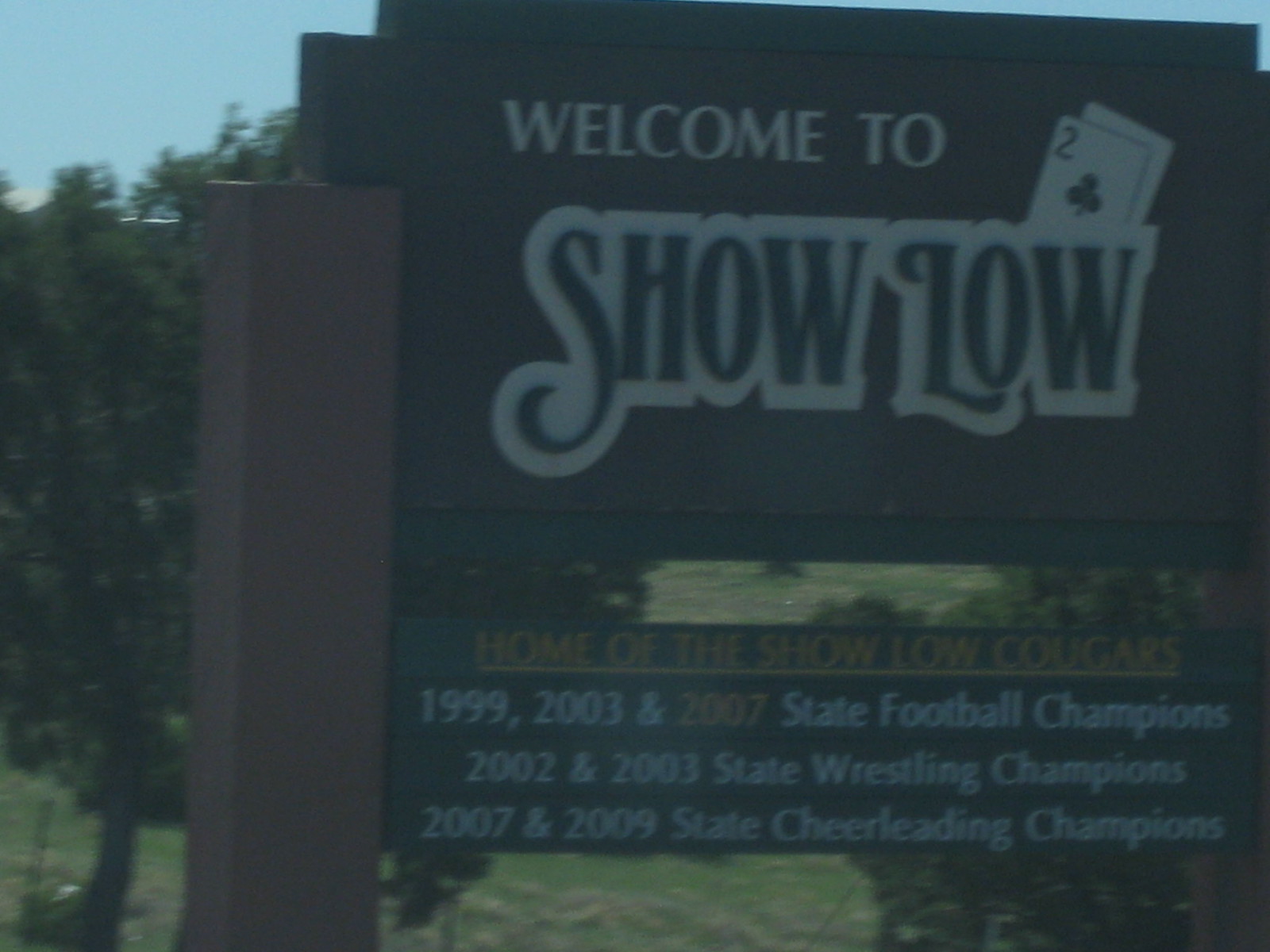This photograph showcases a welcome sign that appears slightly out of focus with suboptimal lighting. The sign is predominantly brown, including its square corner posts. The main surface features white lettering reading "Welcome to Show Low," with the word "Show Low" designed in a distinct font resembling a potential Western or casino style. Intriguingly, behind the word "Low," specifically behind the letter 'W,' there is a depiction of a 2 of clubs playing card, with the outline of another card partially visible. Below this, the sign highlights local sports achievements in yellow print, stating, "Home of the Show Low Cougars," and listing their accolades: "1999, 2003, and 2007 State Football Champions, 2002 and 2003 State Wrestling Champions, and 2007 and 2009 State Cheerleading Champions." The sign is set against a backdrop of brown ground and a few trees, although the background is somewhat blurred, suggesting the photo may have been taken from a moving vehicle.